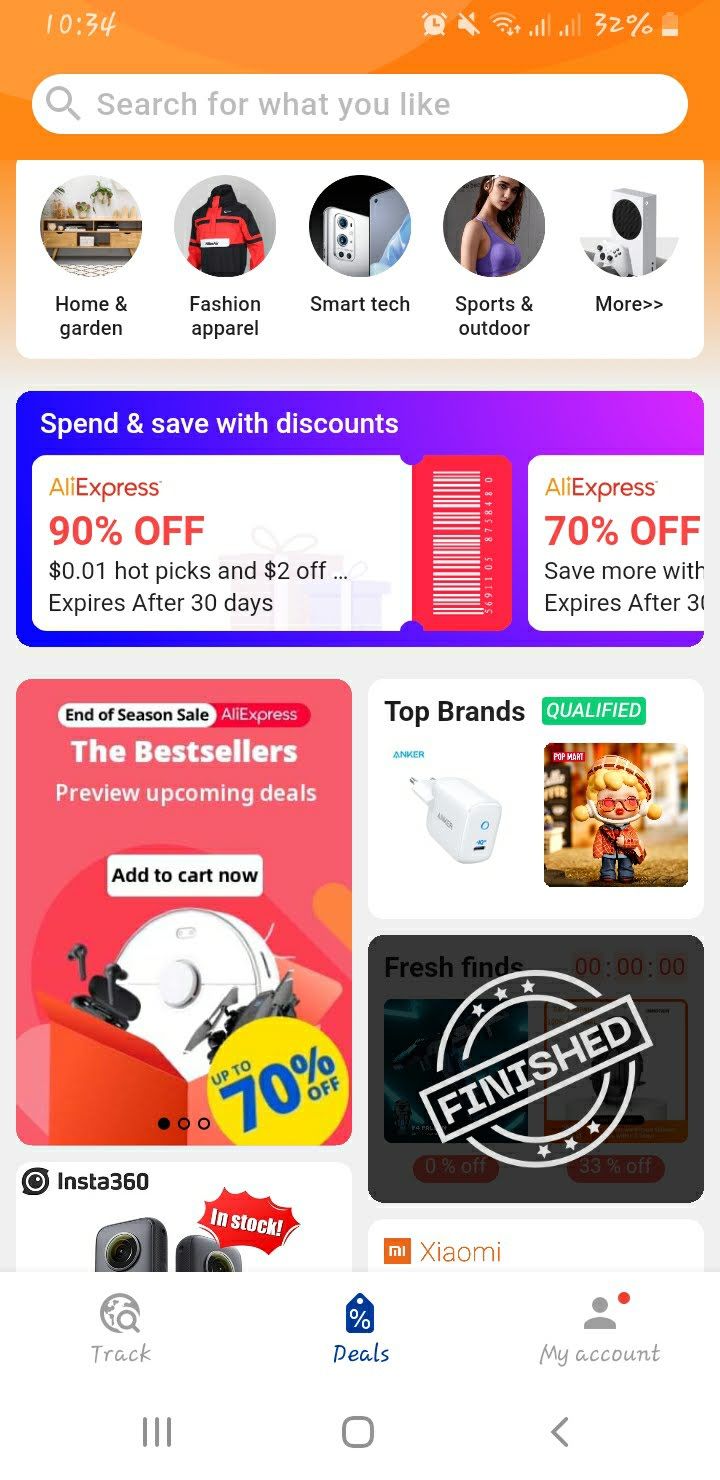This screenshot appears to be from a mobile phone displaying the AliExpress shopping platform. At the top of the screen, there's a search bar to help users find specific products. The interface is categorized into various sections such as Home and Garden, Fashion Apparel, Smart Techs, Sports and Outdoor, and more, indicating that it offers a wide array of products in a single platform. 

Prominent offers like "90% off" and "Hot Picks" are highlighted, enticing users to explore special deals. Scrolling horizontally reveals additional promotional banners, including "End of Season Sale," "Best Sellers," "Preview Upcoming Deals," and "Add to Cart Now." There are images of assorted products including smartphones, a doll, and tech gadgets like an anchor charger and a wall charger under a "Top Brands" section.

The overall appearance of the notification bar includes quirky, almost Comic Sans-like font for the time and battery percentage, adding a unique visual touch to the interface. This platform, likely AliExpress, is known for its extensive range of products, similar to Amazon, and is part of the broader e-commerce market often associated with Chinese goods.